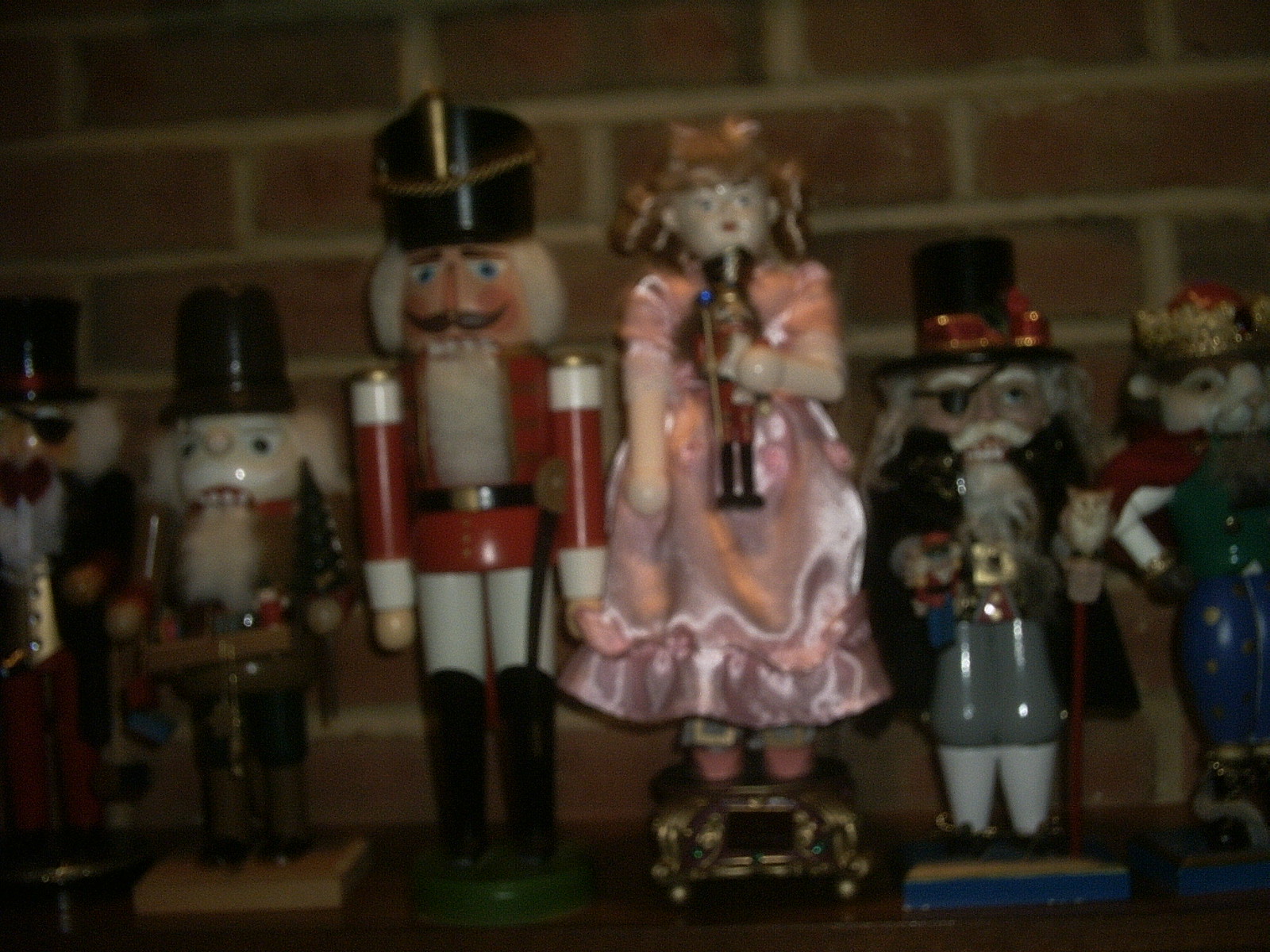This image, though grainy and out of focus, depicts a collection of six distinctive nutcrackers of various shapes and sizes, arranged side by side on what appears to be a dark brown shelf or mantle against a brick wall backdrop. The bricks in the background are different shades of brown, separated by light brown cement.

Starting from the far left, the first nutcracker is only partially visible, adorned in a top hat, an eyepatch over its right eye, white curly hair, a long black tuxedo coat, a red bow tie, a white shirt, and red pants. The second nutcracker has a rounded face, long beard, and wears a tall brown hat. Its image is also highly grainy. The third nutcracker, dressed as a classic soldier, sports a black hat with a chain, a red soldier's outfit, and holds a sword. The fourth nutcracker in the middle is notably different; it depicts a little girl from the Nutcracker Ballet dressed in a pink dress, with curly blonde hair, a pink bow, and white porcelain arms. She's standing on a golden base and holding a smaller typical nutcracker in her hands. The fifth nutcracker is characterized by a black top hat with a Christmas mistletoe in the hat band, which is red with gold trim. It has an eyepatch over its left eye, a mustache, white curly hair, a black cape, gray porcelain pants, white socks, and stands on a blue base while carrying a staff topped with an owl. The sixth and final nutcracker on the far right represents a monkey wearing a crown, a red cape, a green shirt, and blue pants, also set upon a blue base. 

Overall, the nutcrackers range from traditional soldiers to whimsical characters, creating a festive and detailed scene despite the image's lack of clarity.